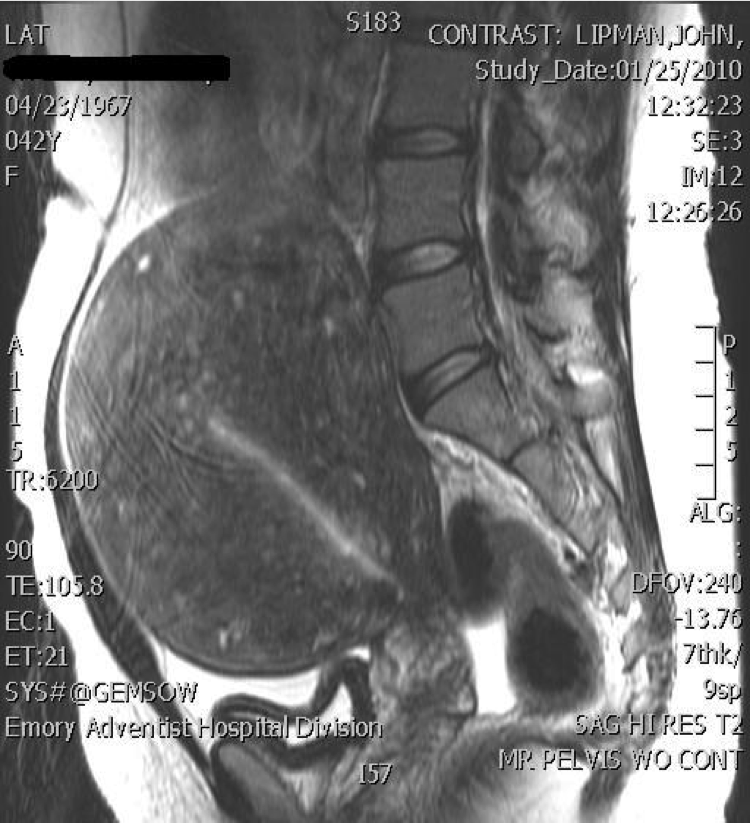The image is a black and white MRI scan of the pelvic region, specifically in a sagittal section, meaning it shows the body from a side view, slicing from front to back. The scan reveals various soft tissue structures, including the spinal column at the top with visible vertebrae and intervertebral discs, the curvature of the sacrum, and the coccyx. The pelvic area also displays an organ that might be the bladder or part of the reproductive system, though not clearly distinguishable. The edges of the pelvis appear rounded, creating a circular shape at the bottom. The MRI scan includes detailed text and numerical information, prominently featuring the patient's name, John Lipman, along with the study date, 1-25-2010, recorded at 12:32:23. Additional data such as a measuring tool and information about the Emory Adventist Hospital Division are also visible on the scan.